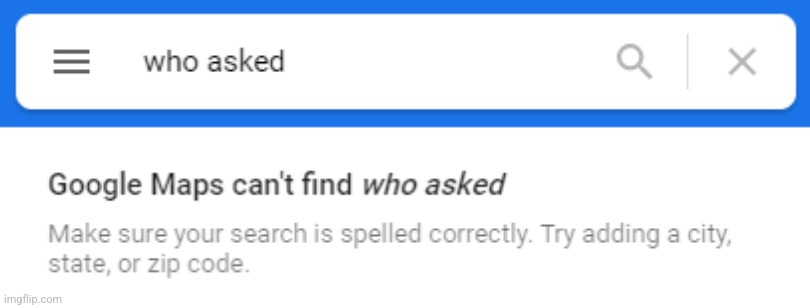A cropped screenshot from a website displaying a Google Maps search query interface. The top section features a white search bar bordered in blue, roughly one centimeter wide. Within the search bar, on the left, there is a menu icon represented by three horizontal lines. The search field contains the black text "who asked?" On the right side of the search bar, there is a search icon depicted by a magnifying glass, a dividing gray line, and a gray 'X'.

Beneath the search bar, the second section has a white background. It prominently displays a bolded and italicized message: "Google Maps can't find who asked." Below this, non-bolded gray text offers suggestions: "Make sure your search is spelled correctly, try adding a city, state, or zip code." At the very bottom, the source of the image is indicated in gray text: "imgflip.com."